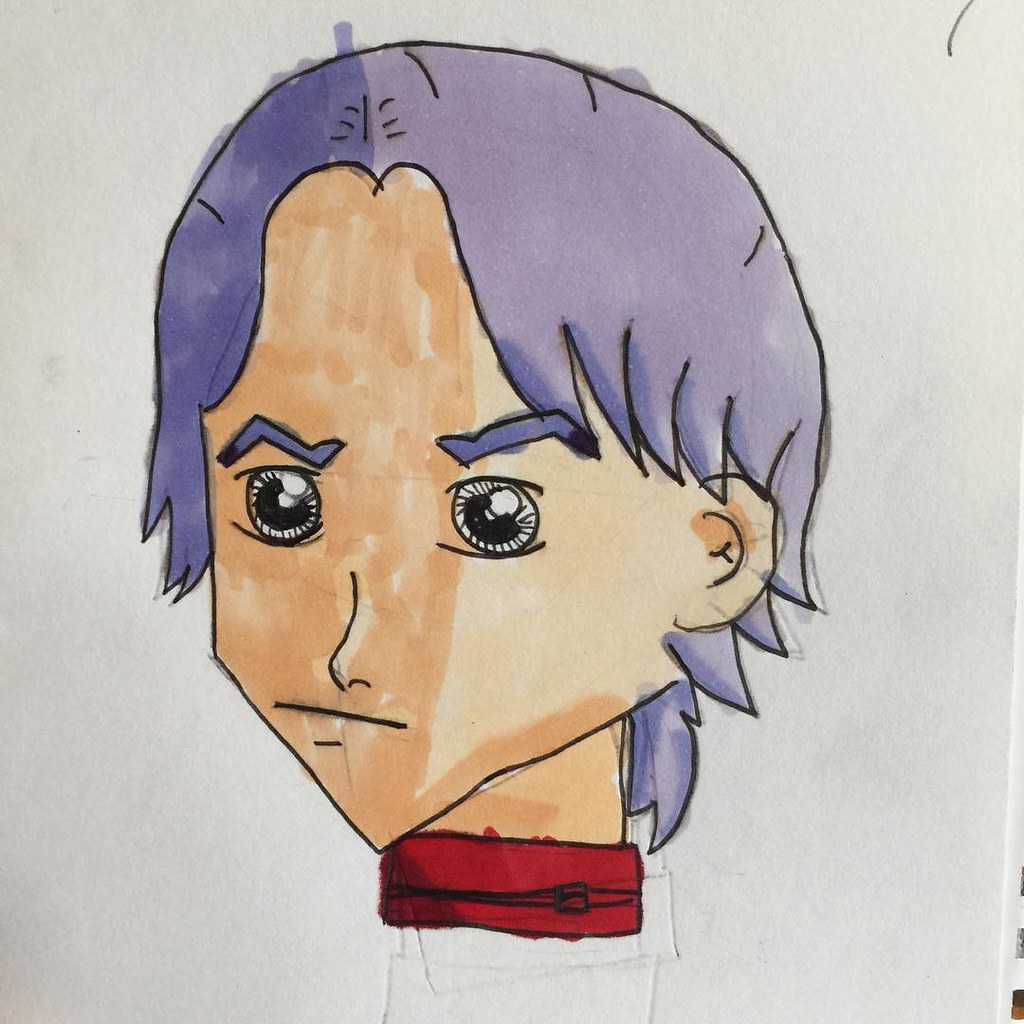This close-up image captures a detailed drawing on a piece of notebook paper, positioned over another piece of paper that reveals spiral notebook holes. The focus of the drawing is on the head and partial neck of an anime-style character, reminiscent of Trunks from Dragon Ball Z. The character features fair skin, lavender-colored shaggy hair that extends to the base of the neck, and matching purple eyebrows. The face is marked by a stern expression, accentuated by black and white eyes, and an angular, pointy chin. The character wears a red collar or band around the neck, adding contrast to the monochromatic facial features. Notably, beneath the final drawing, there are visible erasure marks indicating multiple attempts to perfect the neck and facial details, suggesting a meticulous and iterative drawing process.